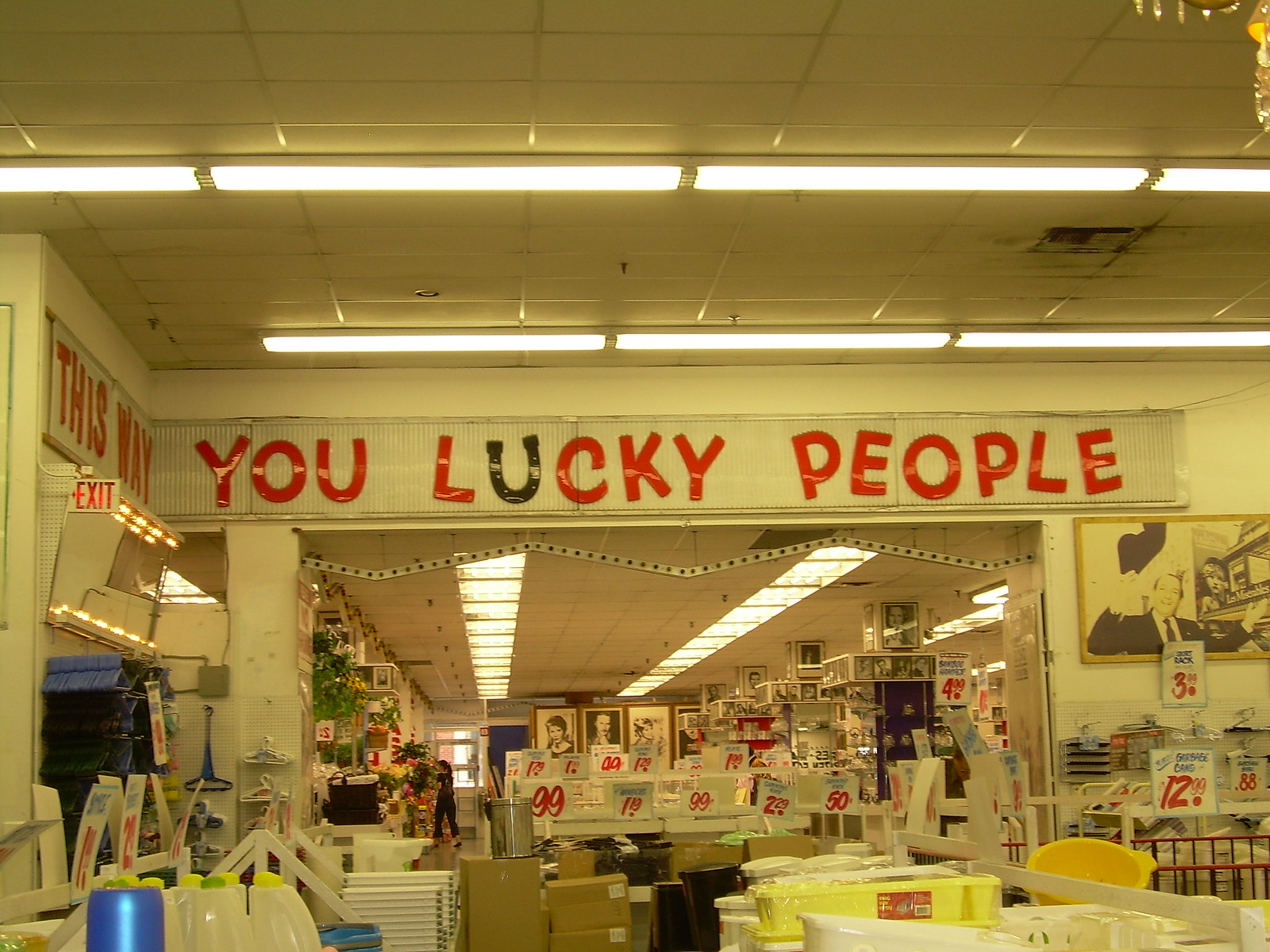A photograph captures a vintage second-hand store with a prominent signage. The main focus is on a large sign mounted on a white background above an opening to another section of the store. The sign's text, "You Lucky People," is in capital letters, with all letters in red except for the letter "U," which stands out in black. These letters are notably large and eye-catching. To the left, another significant sign reads "This Way" in bold letters, directing patrons towards an exit marked by an exit sign. The store's walls are adorned with various signs displaying prices, contributing to a bustling and informative atmosphere. The ceiling is lined with long fluorescent lights, enhancing the nostalgic feel of the store.